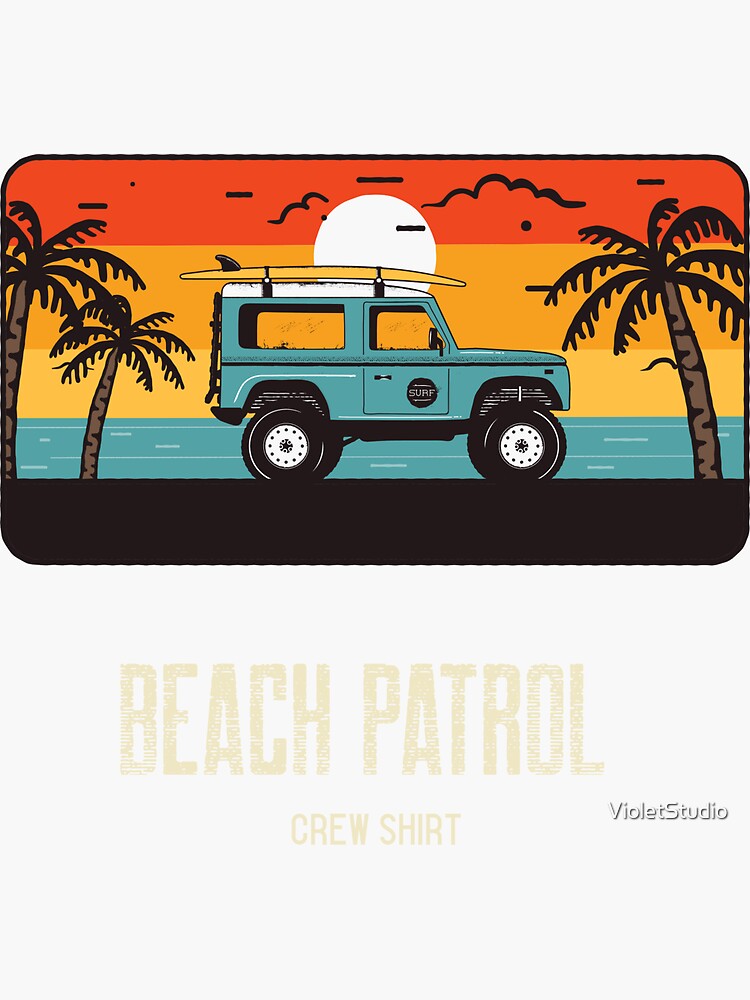The graphic is an illustration of a turquoise Jeep parked in front of a shoreline, with a yellow surfboard attached to its top. Three large, leafy palm trees, bent towards the Jeep, frame the background. A scenic horizon features a setting or rising white sun, casting vibrant hues of orange, yellow, and red across the sky, interspersed with thickly outlined black clouds. The Jeep, adorned with a logo on its side and what appears to be a ladder on the back, faces right towards the water. The bottom of the image has a long black border with the text "Beach Patrol Crew Shirt" and "VLA Studios" beneath the picture, suggesting it is a design for a t-shirt.